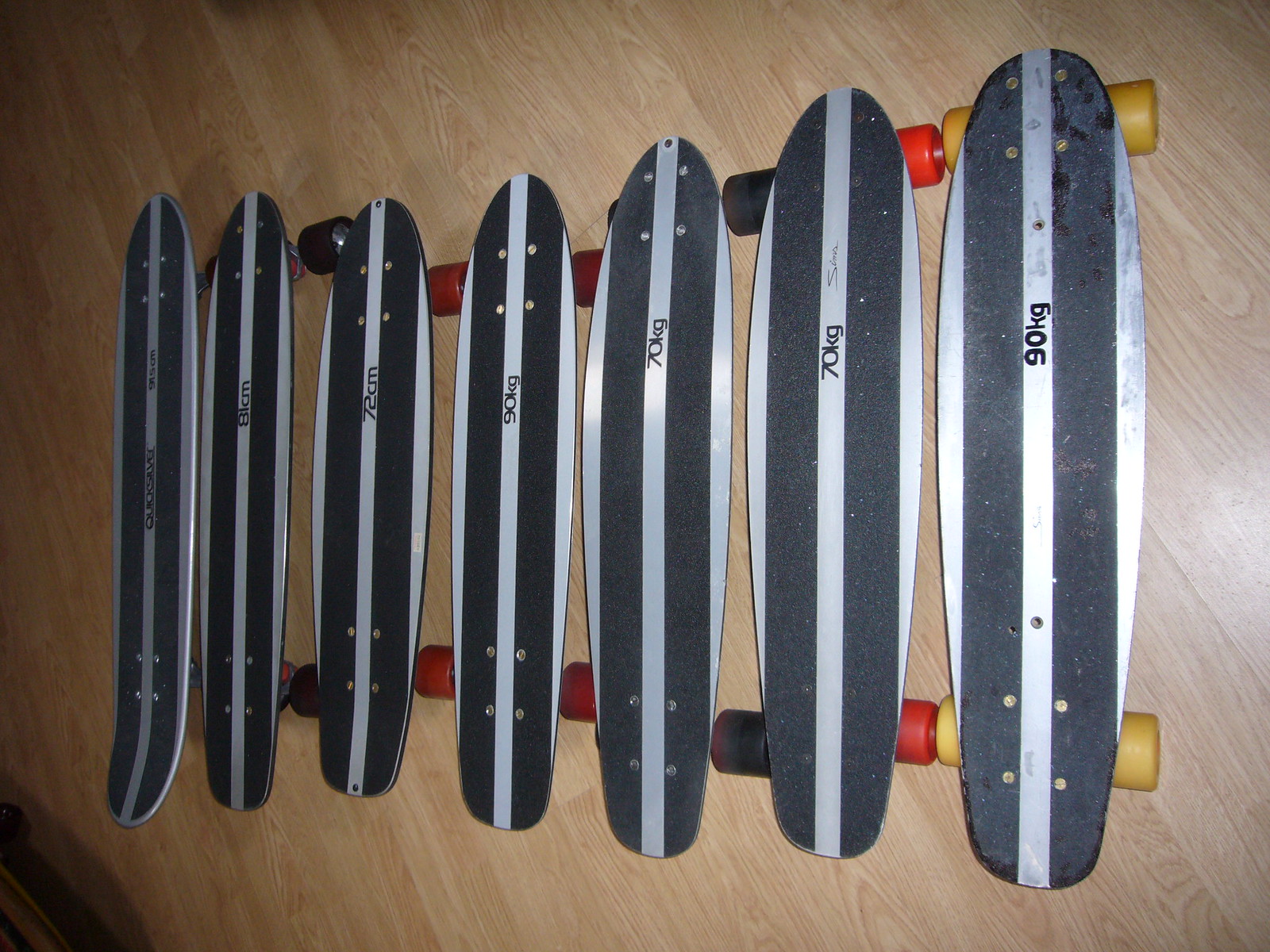The image is a vibrant color photograph capturing eight longboards meticulously lined up side by side on a beach-colored wooden floor. The wooden planks run diagonally from the back left to the back right, complementing the longboard arrangement. The boards, set at a slight diagonal from right to left, are made out of metal and feature two black non-skid grip tape strips with a stainless steel strip running down the center, as well as additional silver strips around the longest edge. They are adorned with visible rivets securing the trucks to the wheels, which vary in color from yellow, black, red, to reddish-orange. The boards closest to the camera on the right display numbers indicating their weight capacities such as 90kg and 70kg, while further boards include variations like 72cm and 81cm. Due to the angle, some numbers and details are not visible. This composition highlights both the uniformity and unique aspects of each longboard, enhanced by the natural wooden background.